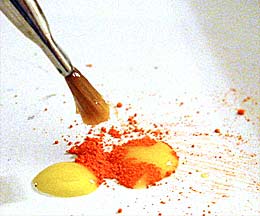This detailed, close-up image, captured on a white background with a faint bluish-grey shadow along the right edge, showcases an untouched artist's palette or sheet of paper. On this pristine canvas lie two prominent, circular blobs of bright yellow paint. Overlaying these vibrant yellow spots, particularly on one of them, is a scattered layer of orange powder, giving the impression that these hues are about to be mixed. The orange granules not only cover parts of the yellow paint but also speckle the white surface around them, suggesting a forthcoming blend of colors.

Dominating the upper left corner, an elegant, medium-sized paintbrush with a silver handle and clean, brown bristles angles diagonally towards the center of the image. The brush’s bristles appear poised above the yellow and orange pigments, ready to mix but not yet touching the colors. The purity of the brush hints at an impending artistic endeavor. The composition's clean lines and distinct colors create a compelling visual, emphasizing the preparation and anticipation of mixing vibrant pigments on the canvas.